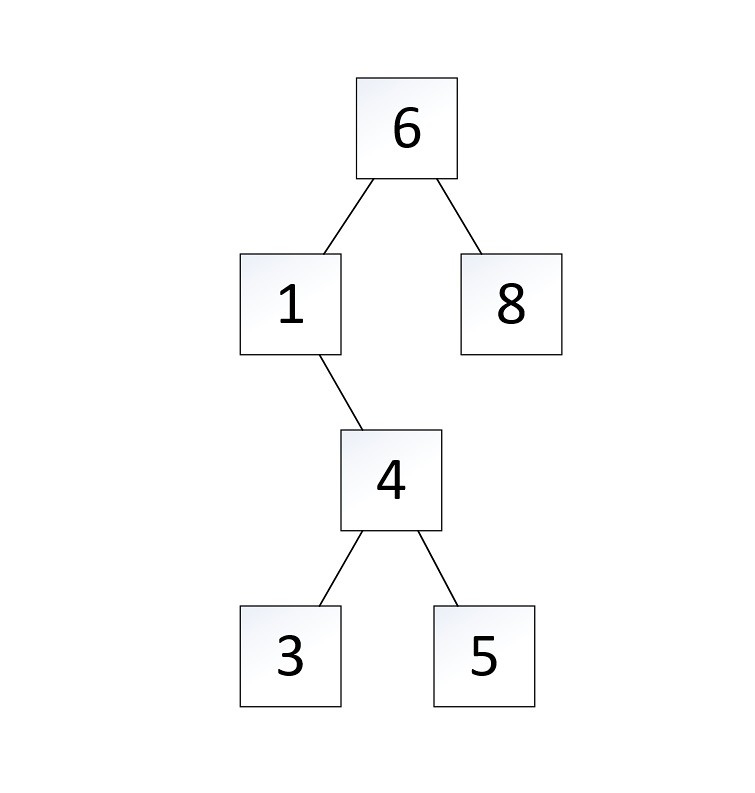This black and white photograph features a detailed number diagram consisting of six squares interconnected by five lines, forming a hierarchical structure. 

At the very top, there is a square marked with the number "6." From this top square, two lines extend downward. The line branching off to the right connects to another square containing the number "8," which has no further connections.

Returning to the top square "6," the line descending to the left leads to a square with the number "1." From this "1" square, a line continues downward to a central square positioned directly below the "6," which holds the number "4."

From the "4" square, two additional lines extend downward. The line veering to the left reaches a square labeled with the number "3," which does not have any further lines.

Lastly, from the "4" square, the line descending to the right connects to a square with the number "5," completing the diagram with no further connections.